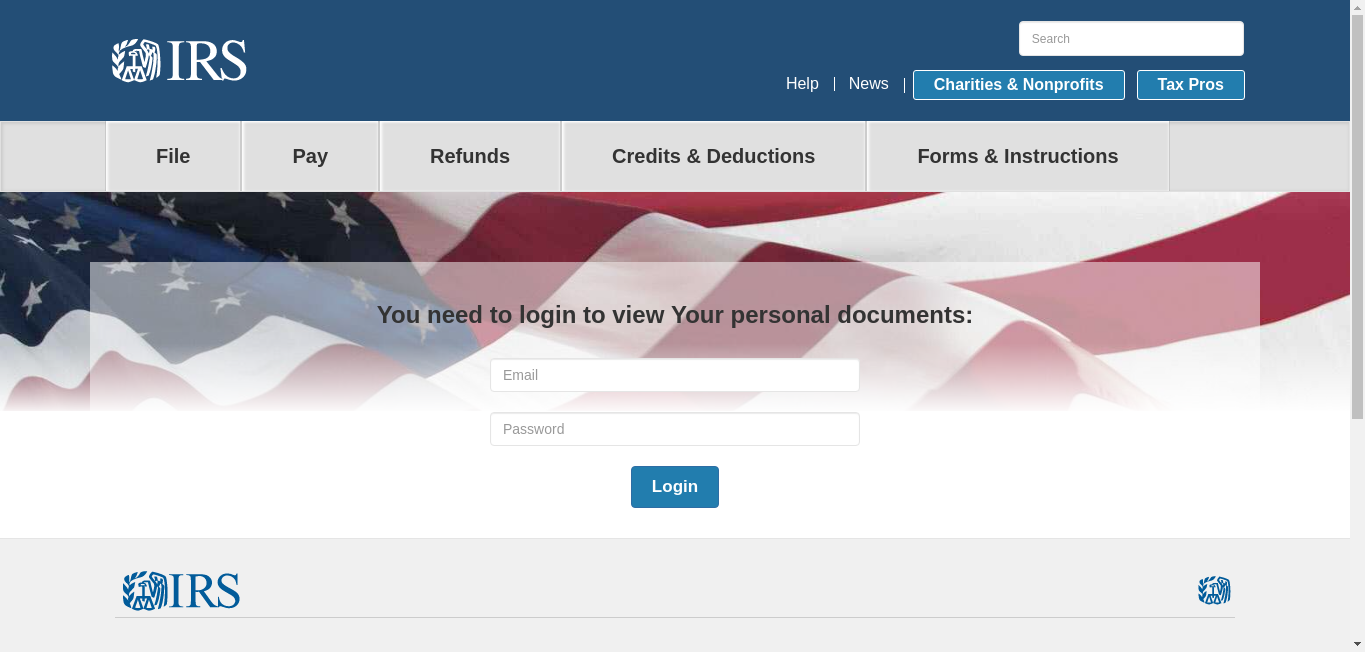This descriptive caption pertains to a screenshot of the IRS website:

At the top of the website is a prominent blue bar stretching across the screen. On the top left within this bar is the IRS logo, showcasing a white vulture holding scales next to the "IRS" acronym. On the top right, a white search bar is visible. Directly beneath the search bar are four buttons arranged in a row: two buttons in white text - "Help" and "News," followed by two blue buttons with white outlines and text - "Charities and Non-Profits" and "Tax Breaks."

Below this section lies a gray navigation menu featuring buttons labeled "File," "Pay," "Refund," "Credits and Deductions," and "Forms and Instructions." Moving further down, there's a banner image adorned with the American flag and a subtle white overlay. The overlay text reads, "You need to log in to view your personal documents." Below this message are two input fields situated one above the other labeled "Email" and "Password." The section concludes with a prominent blue "Log In" button just beneath the input fields.